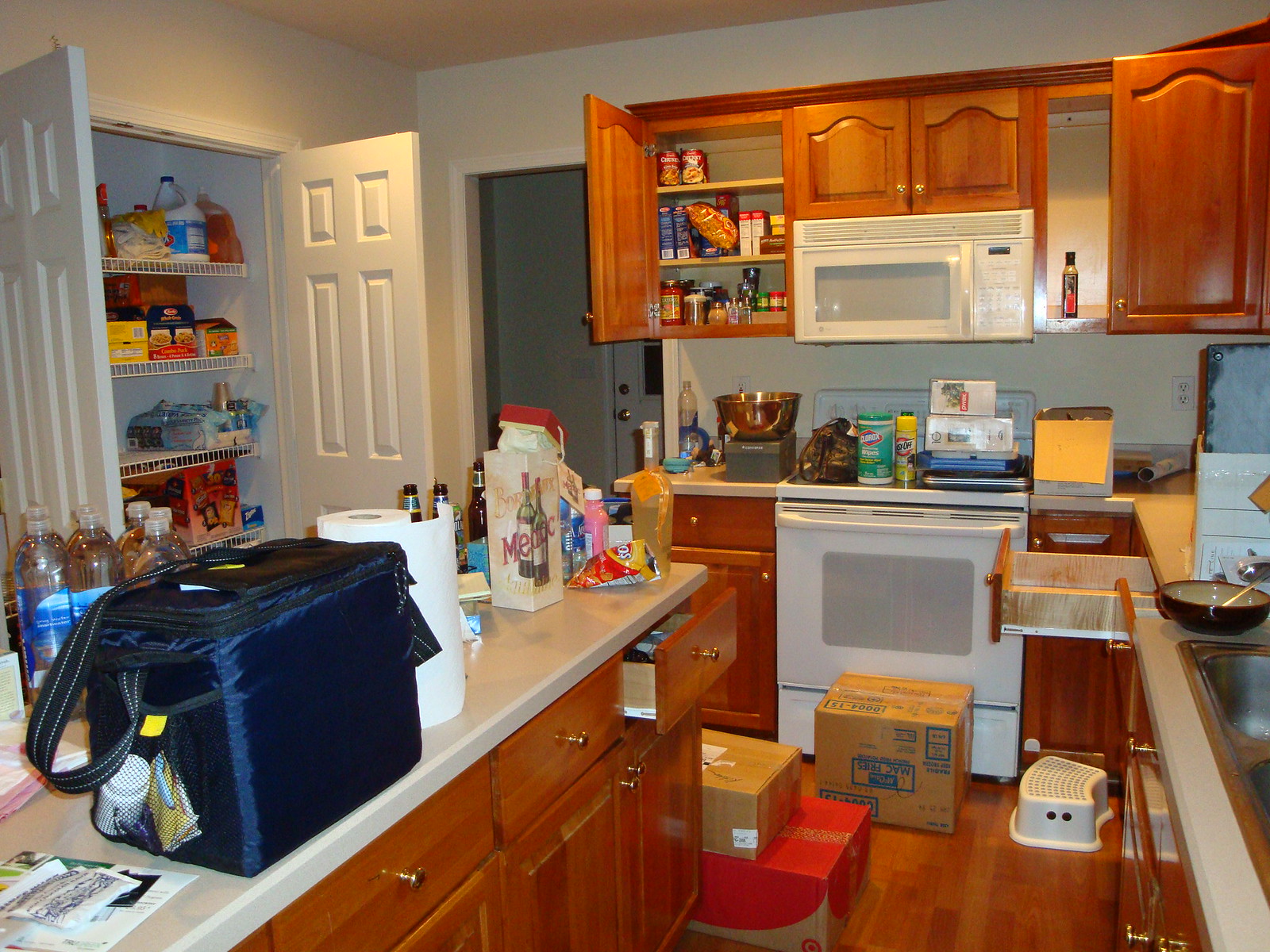A photo captured inside a kitchen, seemingly amidst a move-in process. The kitchen features a wooden floor, scattered with several unpacked boxes. Numerous cabinet and pantry doors are left open, revealing partially filled shelves and compartments. The island counter on the left side of the image is cluttered with an assortment of items, including a bag, rolls of paper towels, various food packets, chips, and bottles. Adjacent to the island are two large doors leading to a pantry, with four visible shelves stocked with additional goods. On the right side, traditional kitchen elements such as cabinets and appliances are visible; the far-right corner houses a barely visible sink. The cabinets are in varying stages of being filled, some open. Meanwhile, the stove top is crowded with miscellaneous items, including a container of Clorox wipes and other stacked objects, all indicative of a busy and ongoing move-in effort.